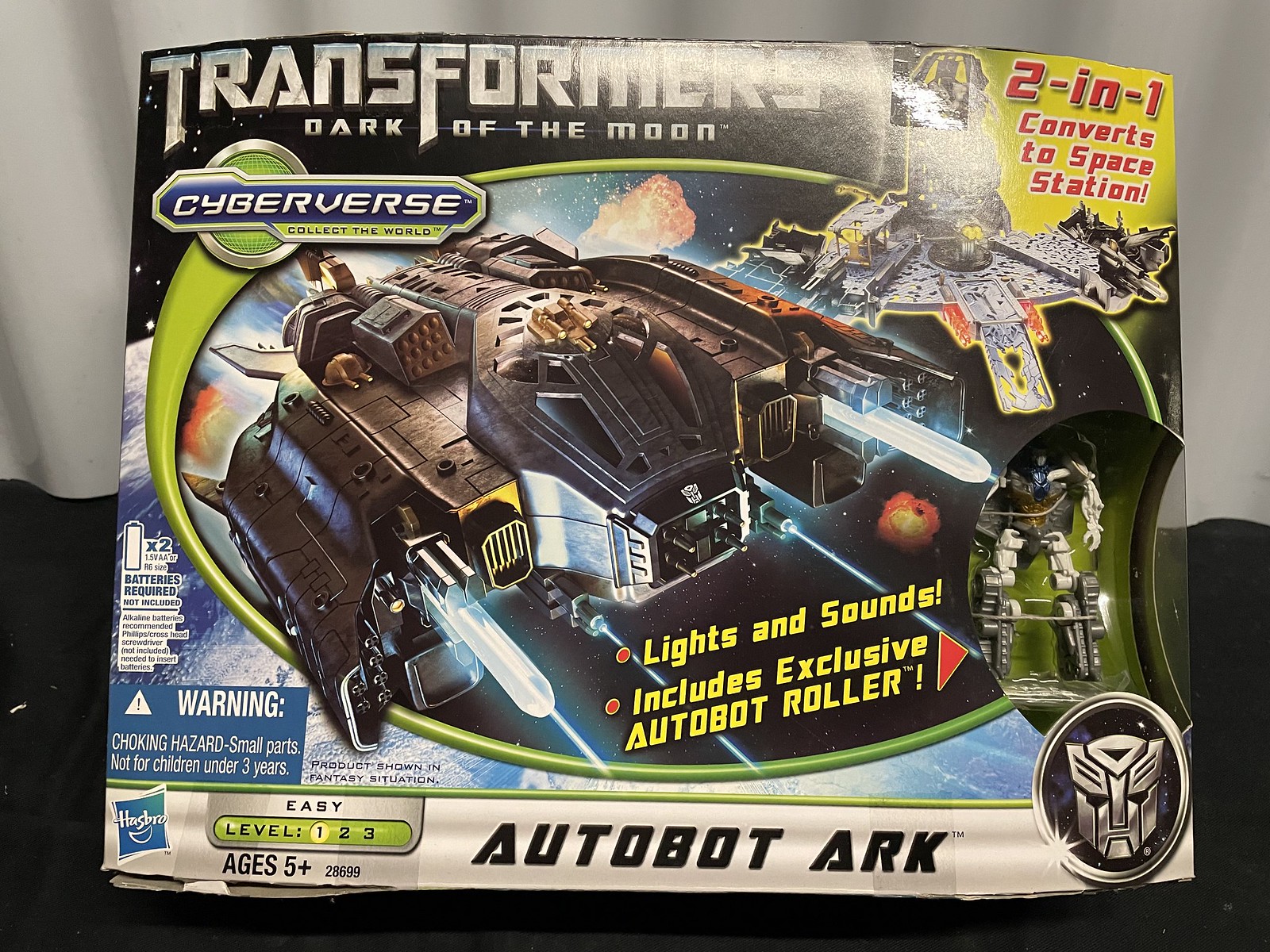This detailed photograph captures the packaging of a vintage Transformers toy from the "Dark of the Moon" series, specifically the "Cyberverse" line. The vibrant box prominently features the title "Transformers, Dark of the Moon, Cyberverse, Collect the World" at the top. Centrally, there is a vivid illustration of the actual toy, the Autobot Arc, depicted as a large spacecraft shooting lasers. Beside this, a yellow burst in the top-right corner announces the toy's "2-in-1" feature, highlighting its transformation ability into a space station, with an image of this alternate configuration provided for comparison.

A cutout window on the right side reveals the exclusive Autobot Roller, a small figure included with the set. Additional details in yellow text emphasize "Lights and Sounds" capabilities. The lower left corner of the package displays the Hasbro logo, along with an age recommendation of "5 and up" and a difficulty rating of "Level 1 out of 3," indicating that the toy is easy to use. There's also a note specifying the requirement of two AA batteries, inferred from the battery image shown. The design style of the packaging is consistent with photographic representational realism, presenting a clear and enticing view of the toy inside.